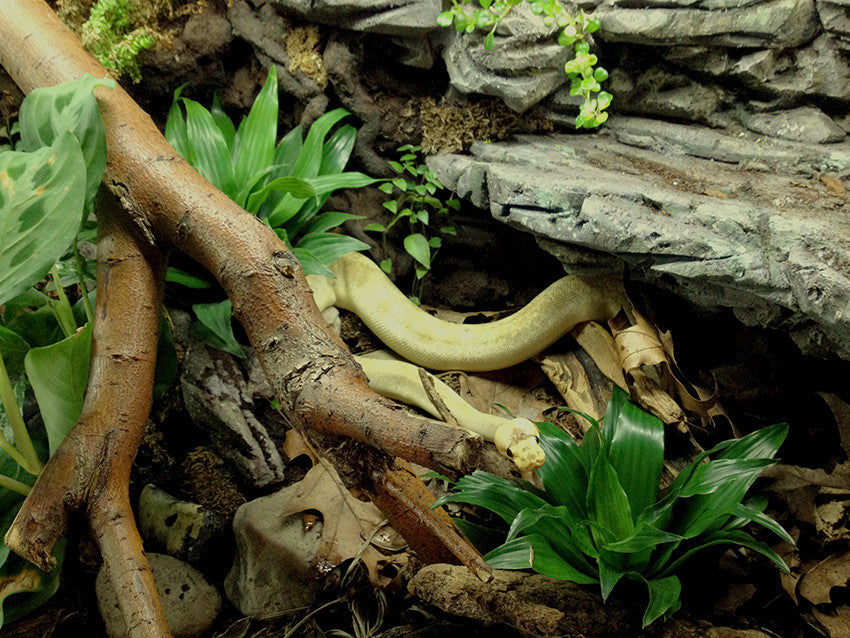The photograph captures a close-up view of a yellow snake partially hidden among the branches and rocks. The snake's face is positioned toward the lower right of the image, with its small black eyes visible. Its body extends leftward before curving upwards and then back to the right, disappearing under a gray, column-like rock formation resembling a shelf. In front of the snake, a green plant with long, slender leaves is prominently visible. To the left is a thick brown branch accompanied by plants with similar thick leaves. The background is cluttered with brown dirt, more branches, dried leaves, stones, and moss, some of which appears dried and some fresh. A creeper with small circular green leaves can be seen trailing down from the top of the image. The overall scene gives the impression of an underbrush habitat where the snake blends into its complex, natural surroundings.